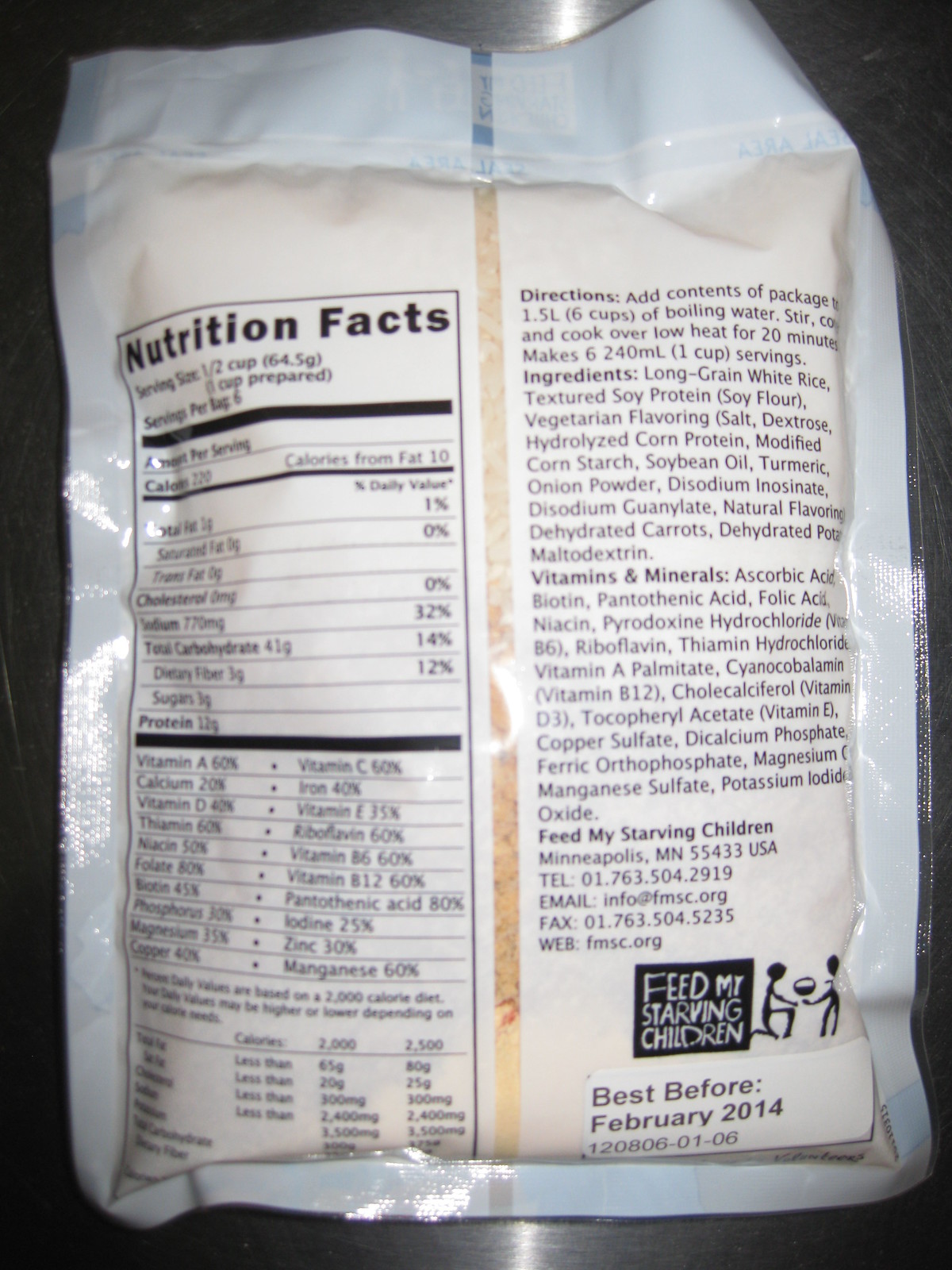The photograph showcases the back of a white, slightly transparent plastic package, containing dried grain material. The text on the package is black, and prominent details include a pull tab positioned towards one side, which reveals nutritional facts when opened. On the opposite side, there are clear instructions for preparation, a comprehensive list of ingredients, and information about vitamins and minerals included in the meal. The package prominently displays the business name "Feed My Starving Children," along with their city, state, and zip code, phone number, email address, fax number, and web link. Additionally, a small black and white logo of the organization features white text in a black square, depicting a kneeling figure and another stick figure with extended arms holding a bowl. A conspicuous sticker on the bag indicates the best before date as February 2014, followed by a series of numbers. The packaging rests on a black, textured, reflective countertop.